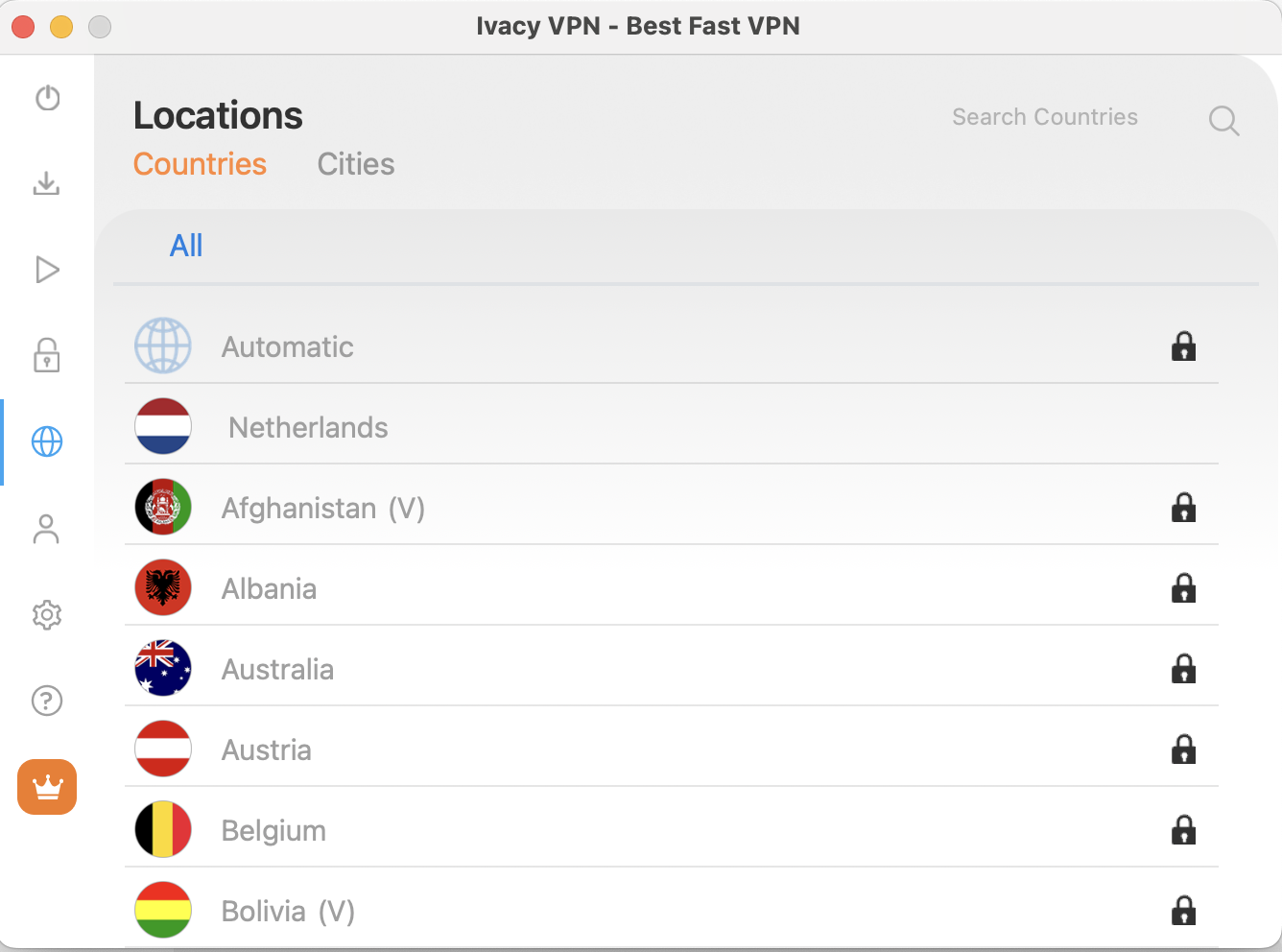**Caption:**

In the center of the screen, the product Avacy VPN is showcased prominently with a description claiming it as the "best fast VPN." The top left corner features three colored circles: red, orange, and gray. The main background of the interface is predominantly gray, with a vertical array of icons aligned on the left side. Beyond these icons, a series of countries is displayed with their flags enclosed in circles.

At the top of the country list is "Automatic" with a lock icon on the right indicating security. Below are countries like the Netherlands (unlocked), Afghanistan (locked), Albania (locked), Australia (locked), Belgium (locked), and Bolivia (locked), among possibly others.

The icons on the left-hand side include:
- A power on/off icon,
- A download icon,
- A play icon,
- A lock icon,
- A globe or country icon,
- A person profile icon,
- A cogwheel for settings,
- And a question mark enclosed in a circle for help.

At the very bottom, an icon of a white crown within an orange square with rounded corners is visible, whose precise function is unclear.